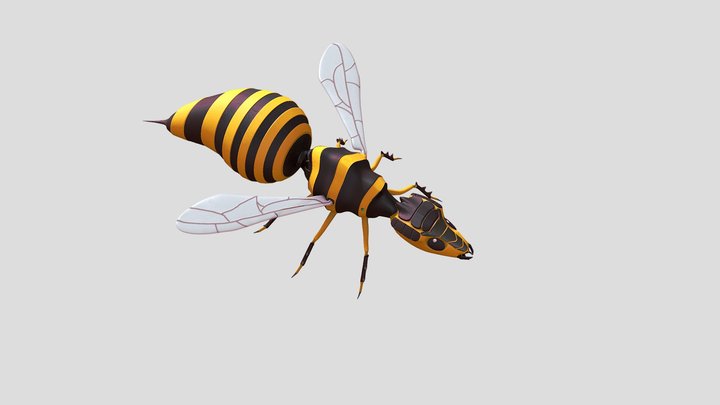This highly detailed and visually striking image showcases a computer-generated yellow jacket or hornet against a plain gray background. The insect features distinct black and yellow stripes running along its body, from head to its large, stinger-equipped abdomen. The head, shaped somewhat like a V, sports black stripes and mechanical-like fangs at the front, enhancing its intimidating look. Its transparent wings, with off-white veins resembling brown cracks, add to the complexity of the design, as do its six yellow, spiked legs. The overall appearance, with its mechanical and inorganic detailing, reveals the insect to be an AI-generated miniature robot rather than an organic creature.